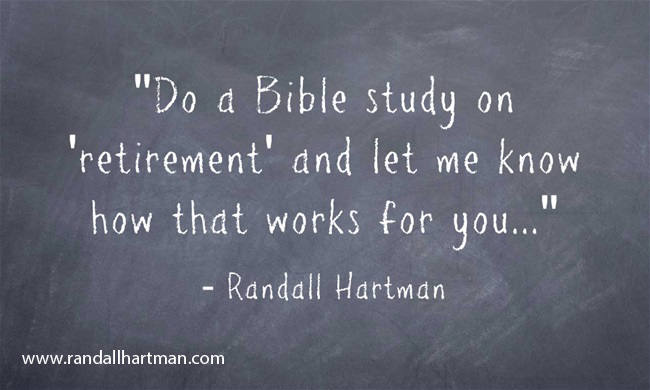The image features a Christian-related quote rendered in a chalkboard style. The quote reads, "Do a Bible study on 'retirement' and let me know how that works for you..." followed by a parentheses and the attribution "Randall Hartman" underneath. The text is presented in white chalkboard-style font on a gray background designed to mimic a well-worn chalkboard, complete with eraser marks prominently visible where the text is located. The surrounding areas of the background are consistently gray. In the bottom left-hand corner, the URL "www.randallhartman.com" is displayed in white Arial font. The entire graphic appears to be computer-generated, with typed text rather than handwritten, and the lighting is evenly distributed across the entire image, contributing to its clean and polished appearance.